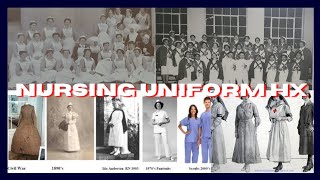The image is a small rectangular collage showcasing the evolution of nursing uniforms from older times to the present. At the top, there are two black-and-white photos of graduating nursing classes in front of a building; the nurses are dressed in traditional uniforms with white aprons and small white hats. Across the middle of the image, in bold white text with a red border, it reads "Nursing Uniform HX," indicating the historical progression of nursing attire. Along the bottom, there are at least nine images of women, each wearing a different style of nursing dress, illustrating the changes in uniforms from the 1800s to today. The grey blocks and side of the building in the background further emphasize the historical context of the collage.